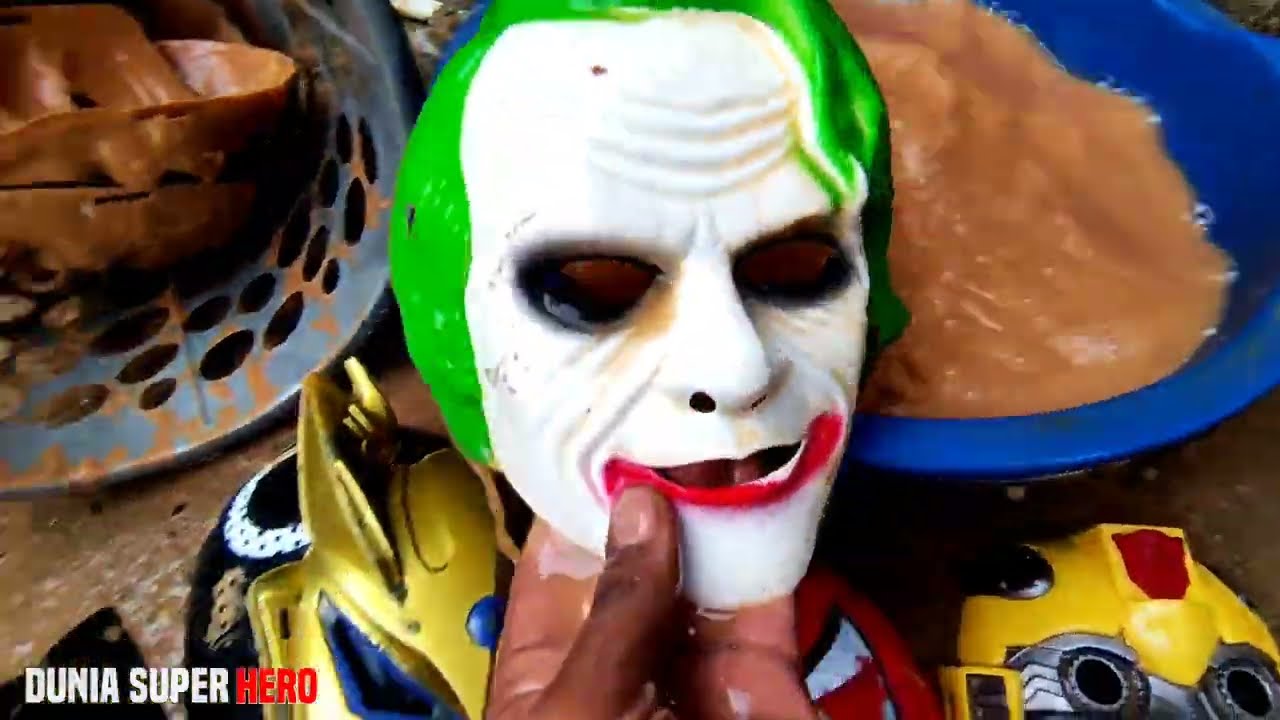In this detailed image, a black artist, identifiable by their paint-splattered hand with short fingernails, is holding a small, intricately designed Joker mask. The mask, predominantly white with no eyes, features lime green hair, a red mouth, and a black, smoky eyeliner effect, reminiscent of the Joker from the Batman movie. It appears to be a mask, likely intended to be worn. 

Surrounding this main focal point are various elements and objects linked to the artist's workspace. On the bottom left corner, a logo reads "Dunia Superhero," with "Dunia Super" in white and "hero" in red, all in capital letters. Also on the bottom right of the image, there is another mask, yellow with silver eyes and a red mouth, resembling a bumblebee in its color scheme. To the left, another sculpture can be seen with vivid gold and blue colors, and blue and black eyes, backed by a black and white section. 

In the top left corner, there's a blue plate with black dots, while the top right corner features a blue plastic bowl filled with a glossy brown clay-like substance, appearing caramel in color. Additional exploratory elements include another indistinct red mask with visible white stripes and a likely mold-making material positioned underneath the Joker mask and the artist's hand. The overall scene is lively, showcasing the artist’s mixed media workspace and their detailed, colorful creations.